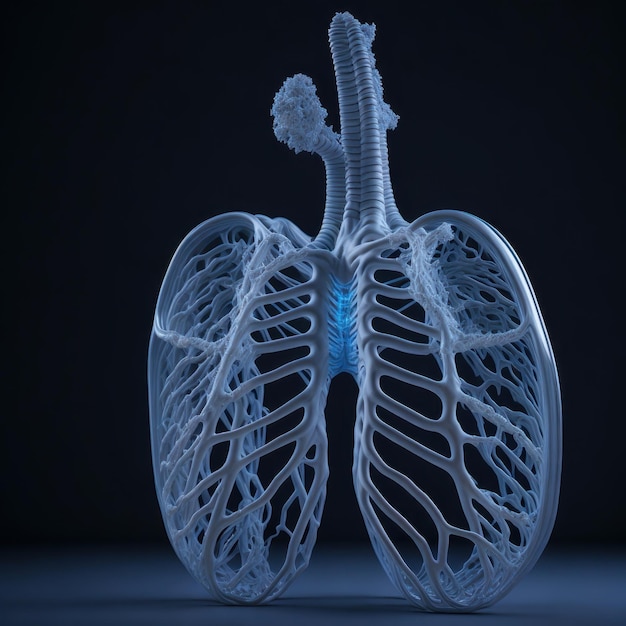This detailed image depicts a computer-generated 3D rendering of a human ribcage and lungs in a white and light grayish blue color scheme, with a touch of blue highlighting. Set against a stark black backdrop, the 3D print exhibits exceptional clarity and texture, revealing the intricate anatomy of the bronchial tubes and cilia. The depiction includes the outline of the windpipe and vertebrae, offering a comprehensive view of the respiratory system that appears almost skeletal due to the pristine white coloration. The transparency of the print allows visual access to background details, accentuated by a faint blue haze enhancing the contrast. The central part, where the lungs attach, features a glowing blue patch, further emphasizing the structure. This diagnostic-quality 3D rendering illustrates the complex network within the lungs, making it an invaluable tool for educational and medical purposes, as it permits examination from multiple angles.